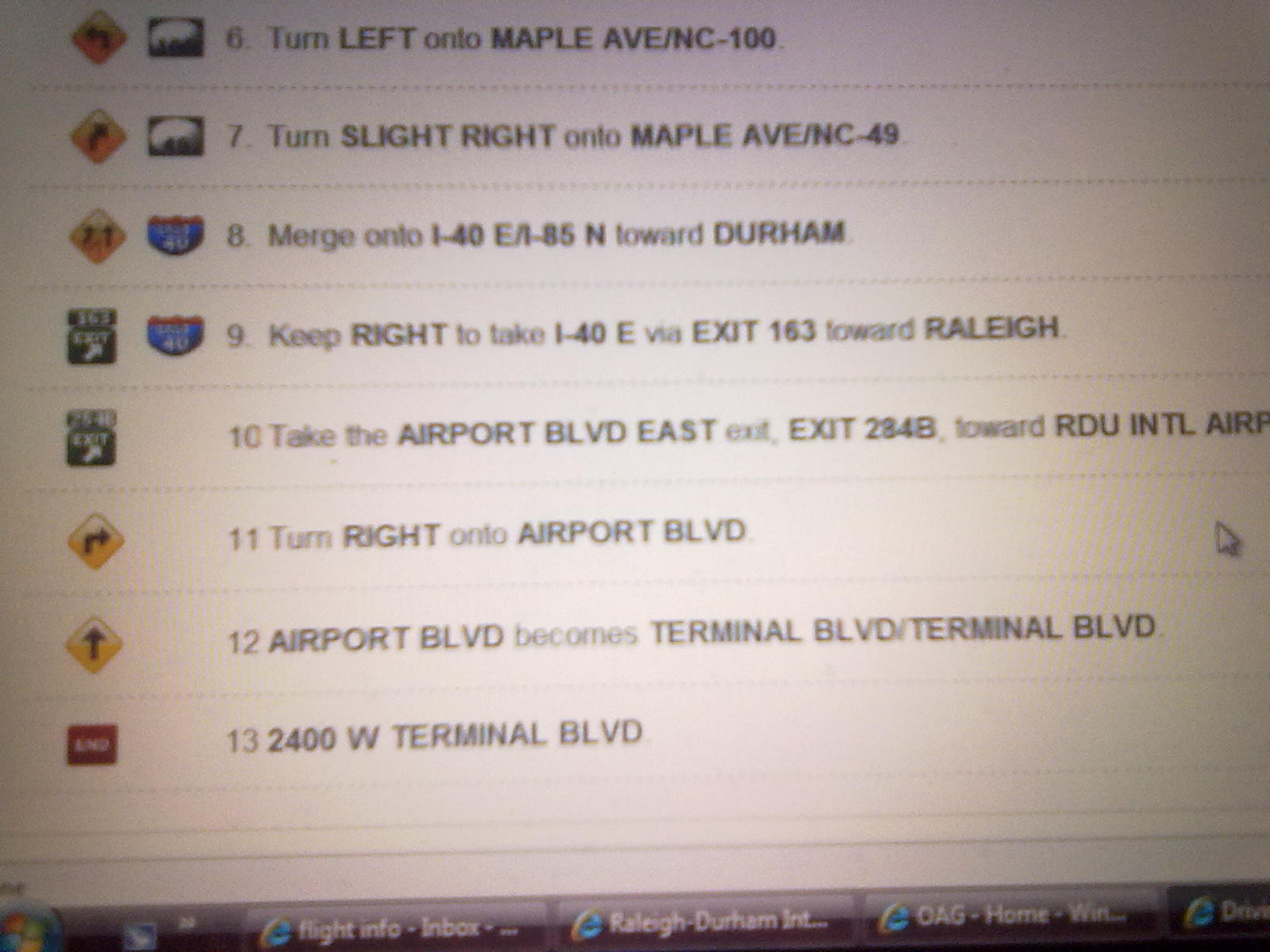This image is a blurry photograph of a computer screen displaying driving directions to an airport terminal, with the directions presented in a map application on Internet Explorer. The visible instructions start from number 6 and continue sequentially through number 13, which is the final destination labeled "2400 West Terminal Boulevard" marked with a red box reading "END." Each step includes detailed instructions such as road names, like Maple Avenue, and directional icons, for instance, a black left arrow on a yellow background. At the bottom of the screen, there are four open Internet Explorer tabs visible.